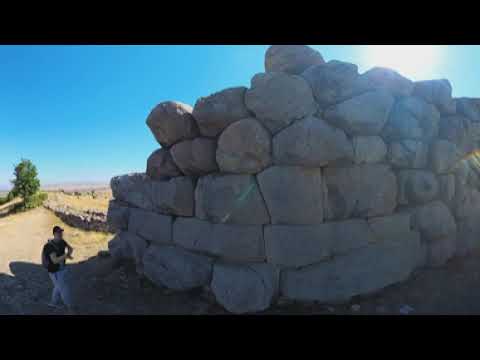This photograph, likely taken in an outdoor setting, captures an impressive formation of stacked rocks, creating a massive, wall-like structure of varied shapes—some nearly rectangular, others more rounded. The striking detail of this image reveals rocks larger than a human, towering and meticulously arranged, suggesting significant effort and perhaps historical importance. The man in the image, walking near the base of the rock wall, provides a sense of scale; he wears a dark short-sleeve t-shirt, light pants, and a baseball cap, and carries a backpack. The terrain appears dry, covered with brown soil and light sandy patches. The sky above is brilliantly clear, a vibrant turquoise blue, with the sun shining brightly from the right, casting deep shadows that offer cool shade against the sun's intense light. In the background, a lush green tree or large bush stands out amid the arid landscape, enhancing the natural beauty of this scene. Despite its slight blurriness and curved framing with black horizontal lines at the top and bottom, the photograph leaves a powerful impression of the juxtaposition between human and natural elements.